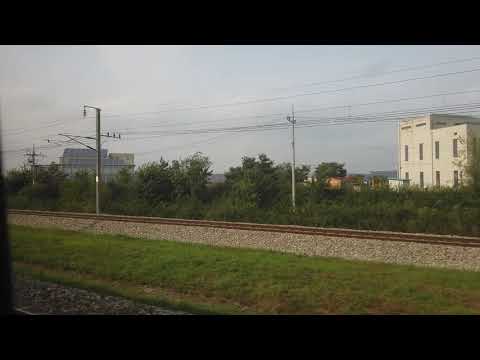This image is a vertically oriented rectangular photograph framed by horizontal black stripes at the top and bottom. Central to the scene are brown steel railroad tracks running horizontally from just below the center on the right to just below the center on the left, nestled within a gravelly area. On either side of the tracks, short green grass is visible in the foreground, transitioning into taller grass and green shrubbery. In the background, there's a row of small green trees. Several telephone poles, each with power lines stretching across the gray, cloudy sky, line the tracks. To the right, behind the bushes, stands a small white two-story concrete building. To the left, another building with a gray roof, possibly agricultural, can be faintly seen behind one of the telephone poles. The scene is void of people and text, presenting a tranquil, deserted railway environment.